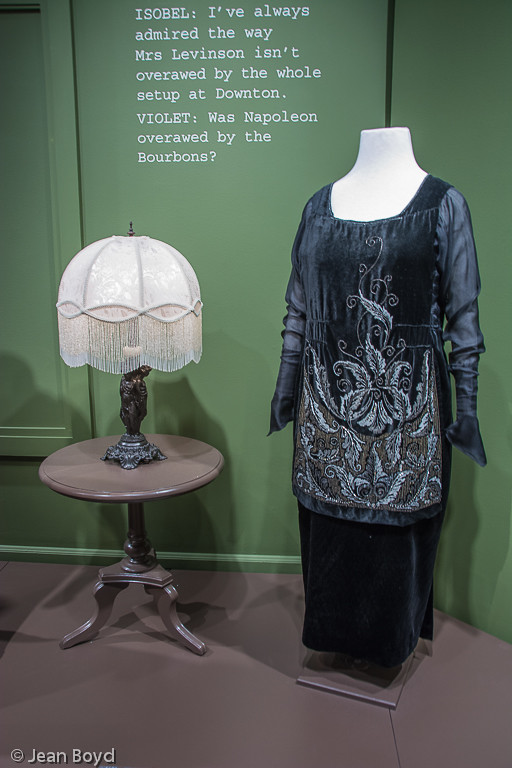The image is a museum display set against an olive green wall with a wooden brown floor. On the left, there is a small, round coffee table with a black, ornate lamp in the center. The lamp has a white, dome-shaped lampshade decorated with numerous little tassels hanging from its edge, resembling a jellyfish. On the right side stands a headless white mannequin dressed in a purple floor-length gown adorned with intricate leaf patterns on the apron part of the dress. In the upper middle part of the image, the wall has white text that reads: "Isobel, I've always admired the way Mrs. Levinson isn't overawed by the whole setup at Downton. Violet, was Napoleon overawed by the Bourbons?" In the bottom left corner, the text "Copyright Gene Boyd" is visible.